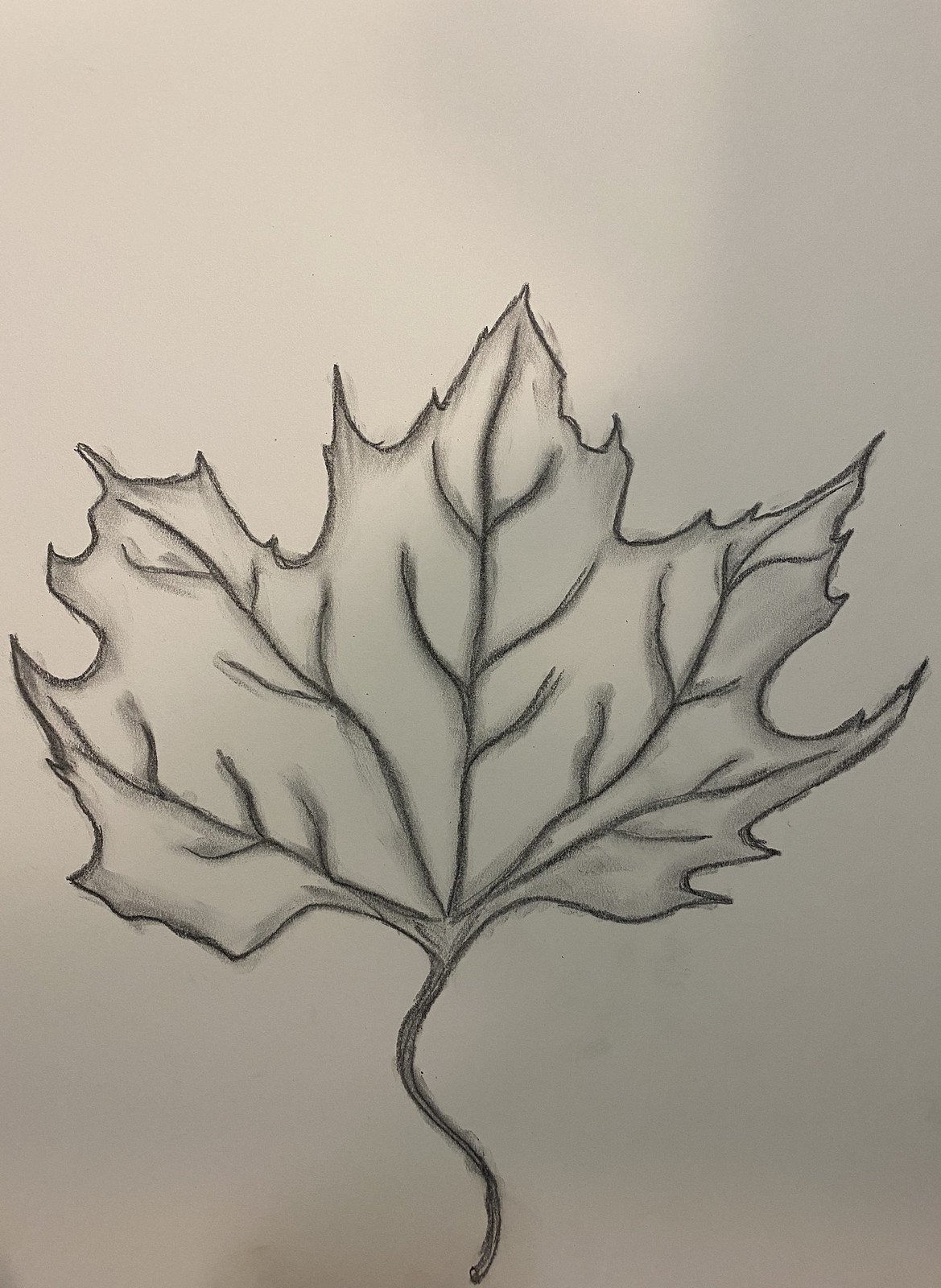This vertical rectangular image captures a beige-colored background of a piece of paper adorned with a meticulously crafted pencil sketch. The sketch, rendered in a sepia tone with a bold black outline, depicts a single, intricate maple leaf that occupies approximately half of the paper. The leaf stretches horizontally from left to right, showcasing its deeply carved crevices and detailed structure. The veins of the leaf are prominently shadowed, adding depth and realism to the drawing. Below the leaf, the stem curls gracefully into an S-shape, adding an elegant touch to the composition. The entire leaf is shaded lightly, allowing the stark and dark outline to stand out, emphasizing the delicate artistry of the sketch.